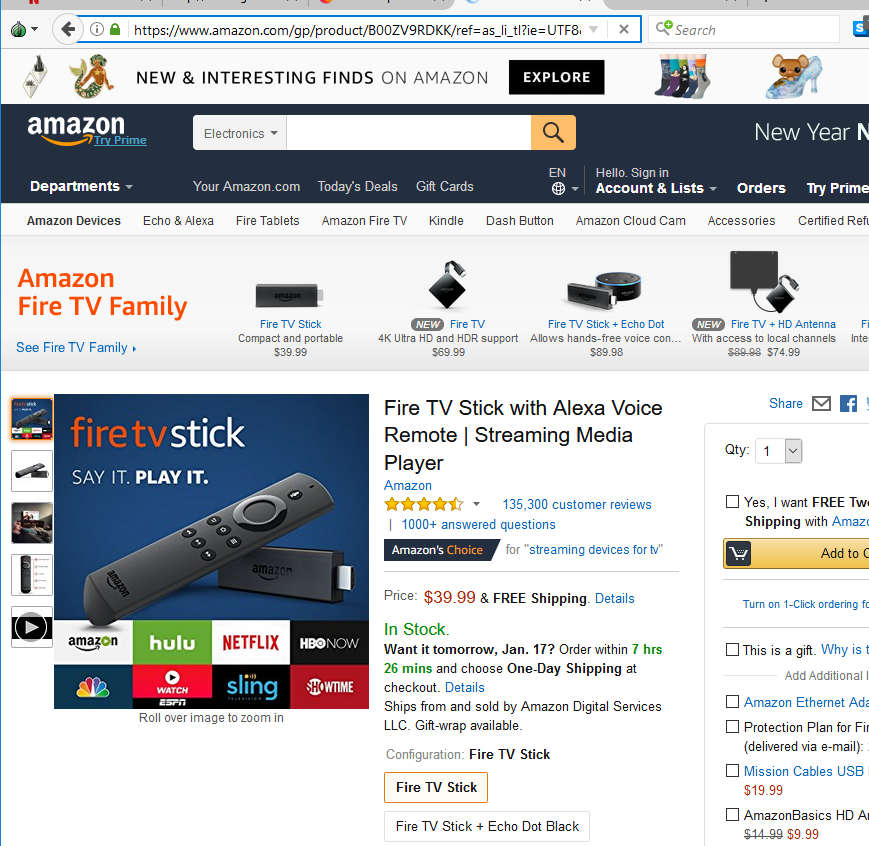A detailed screen capture of half of the Amazon homepage is shown. The familiar color scheme of the Amazon website is immediately noticeable, featuring a white banner at the top followed by a black header displaying the white, orange, and blue Amazon logo in the top left corner. To the right of the logo is a gray drop-down menu for selecting categories. Adjacent to this is a prominent white search bar, followed by an orange search button emblazoned with a magnifying glass icon.

On the upper right side of the banner, white text partially visible reads "New Year." The typical Amazon headings are also present: "Departments," "Your Amazon.com," "Today's Deals," "Gift Cards," "English" as a language option, and then further headings like "Hello, Sign In," "Accounts and Lists," "Orders," and "Try Prime."

Beneath the main header, a product menu is displayed against a white background, listing categories from left to right including "Amazon devices," "Echo and Alexa," "Fire tablets," and "Amazon Fire TV," among others. In orange lettering on the upper left, it reads "Amazon Fire TV family," highlighting various devices Amazon offers for streaming.

The image prominently features a large blue background on the left part of the product page, displaying an Amazon Fire TV Stick. Bold red text reads "Fire TV," and diagonally across the image from the lower left to the upper right is an image of the Fire TV Stick remote. Beneath the remote, the USB dongle is visible on the right-hand side. Surrounding this central image are smaller icons: on the left are additional images of the device, and along the bottom are logos of various streaming platforms supported by the Fire TV Stick.

In the center, bolded black text announces "Fire TV Stick with Alexa Voice Remote streaming media player," followed by a detailed product description. The price for this device is listed at $39.99. On the right-hand side, partially visible, is the "Add to Basket" section, with the usual supporting text beneath it, offering the user a seamless option to proceed with their purchase.